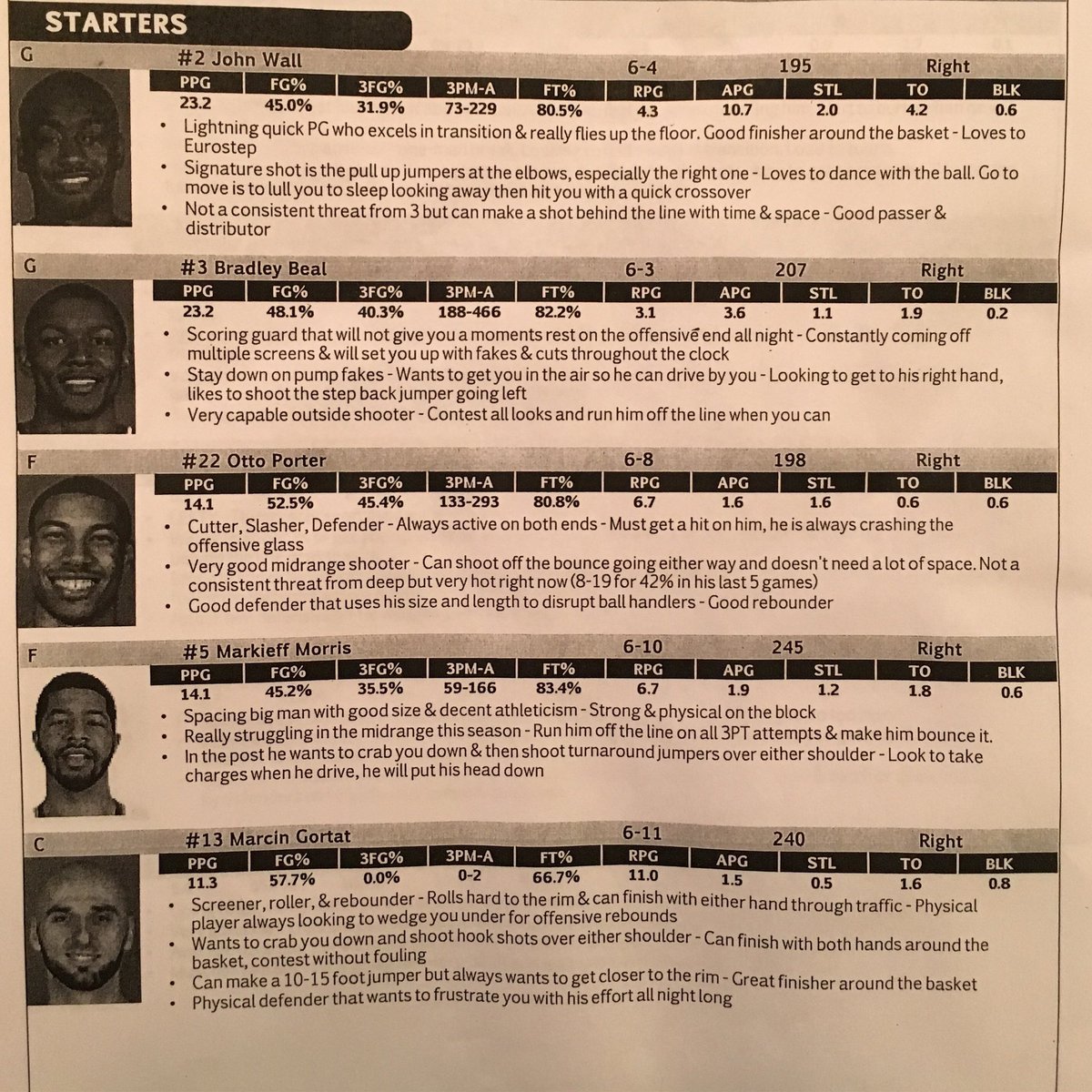This image depicts a light pink page, possibly from a team magazine, showcasing the statistical highlights of five Washington Wizards players for the season. At the top is John Wall, who wore the number 2 jersey. He averaged 23.2 points per game with a field goal percentage of 45% and a three-point shooting percentage of 31.9%.

Next is Bradley Beal, number 3, matching John Wall in scoring with 23.2 points per game. Beal boasted a higher field goal percentage at 48.1% and an impressive 40.3% from beyond the arc.

Below Beal is Otto Porter, the number 22 player. Porter recorded 14.1 points per game, shooting 52.5% from the field and a notable 45.4% from three-point range.

Following Porter is Markieff Morris, identifiable by his number 5 jersey. Morris averaged 14.1 points per game with a field goal percentage of 45.2% and 35.5% from three-point land.

At the bottom is the center, Marcin Gortat, known for his size and stature at 6'11". Gortat averaged 11.3 points per game with a field goal percentage of 57.7%, but did not make any three-point attempts. Additionally, Gortat was a dominant rebounder, pulling down 11 rebounds per game.

The statistics vividly capture the contributions of these key players during their time with the Washington Wizards.